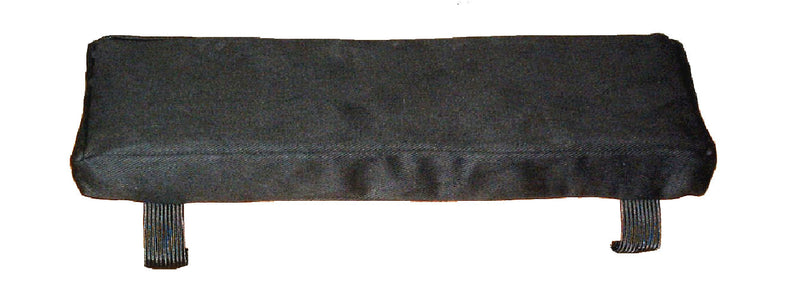The image depicts a cushion resembling a meditation bench, set against a plain white background. The bench is rectangular and narrowly shaped, upholstered in black fabric that slightly reflects light, suggesting the use of flash photography. Measuring approximately 2 to 3 feet in length and no more than 8 inches in width, it appears portable. Below the cushion are two elastic or velcro straps, each about half an inch in width and exhibiting a dual gray color scheme with light gray on top and darker gray on the inseams. These straps hang down freely, curving at the bottom, and aren't attached to anything. Some faint signs of dust and white fur on the fabric indicate that the product may be pre-owned. The image is devoid of any text, pricing, or branding, focusing solely on a detailed visual depiction of the bench.